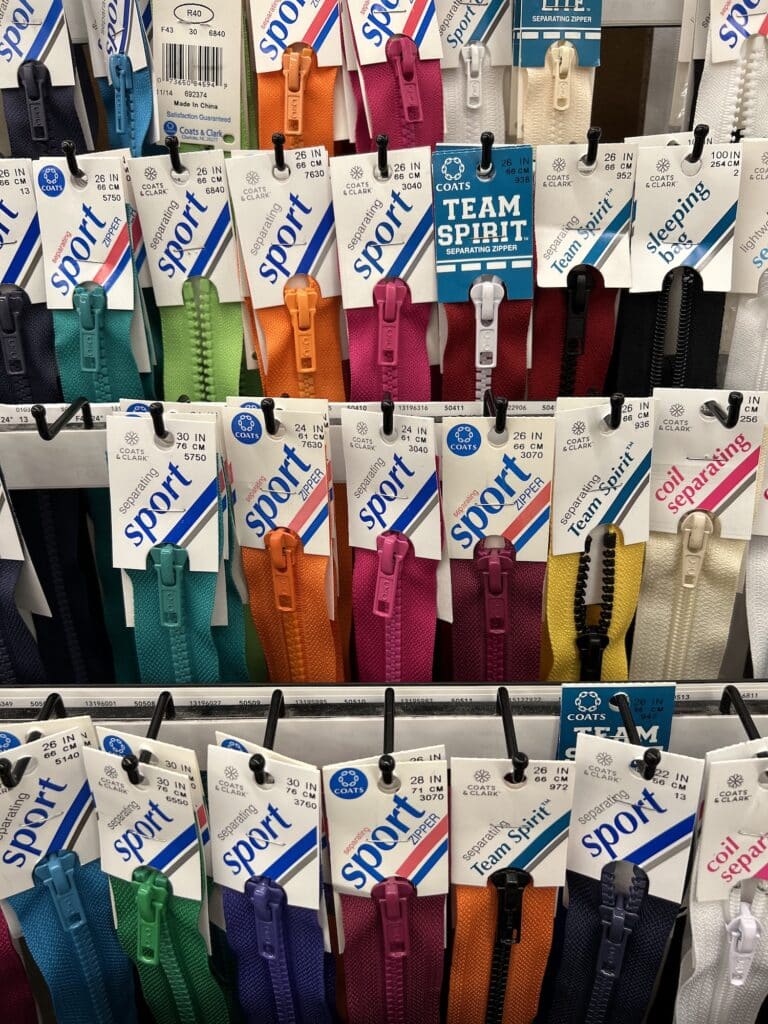This image showcases four well-organized rows of zippers on display in a store, each row suspended from evenly spaced black hooks. The zippers present an array of vibrant colors including teal, various shades of green such as violet green and forest green, orange, pink, maroon, burgundy, black, blue, yellow, cream, white, beige, gray, and different shades of purple from light to dark. Each zipper is affixed to the hooks by their white tags, prominently labeled under brands like Separating Sport and Team Spirit, all produced by Coats and Clark. The detailed arrangement reveals an extensive selection ready for any sewing project.